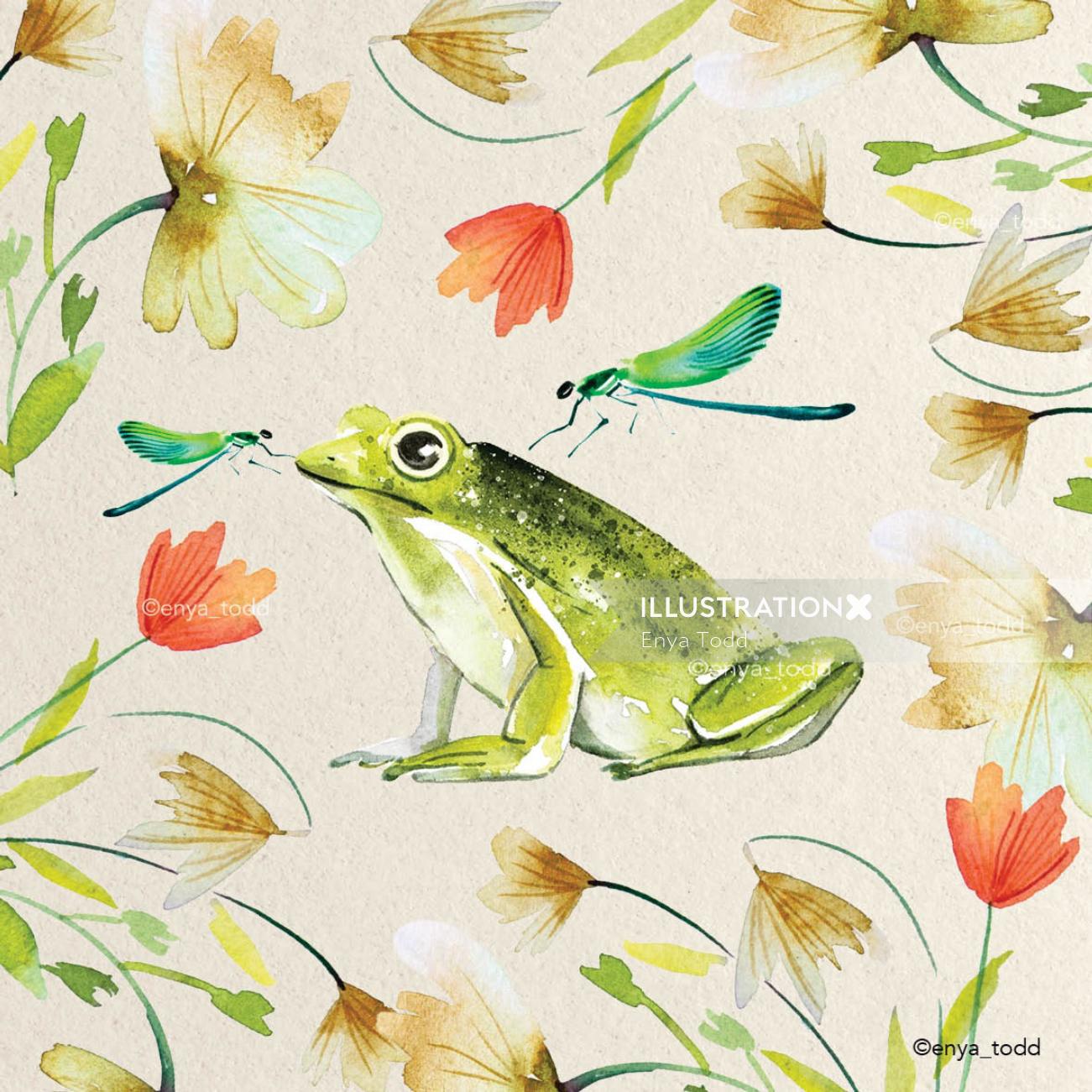The illustration features a green frog with a white belly and a dark green back, centrally positioned on a textured, off-white background that resembles watercolor-style paper. On either side of the frog are two bluish-green dragonflies, one perched on its nose and another hovering near its back. The scene is enriched with a variety of flowers, including white, beige, light red, and pinkish blooms with green stems and leaves, as well as some yellow leaves. The imagery suggests a lush, natural setting with a serene, artistic feel. The right side of the artwork is labeled "Illustration X," accompanied by the artist's signature "Enya Todd" and the website "Enyatod.com." The backdrop's matte texture gives the piece a subtle, wallpaper-like quality.